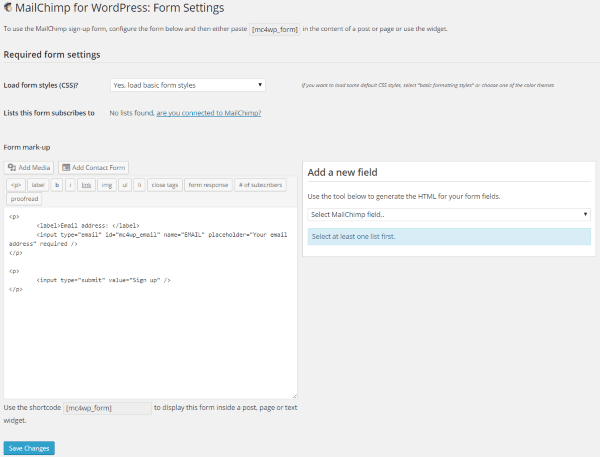The image displays a user interface for configuring form settings in "MailChimp for WordPress." The interface is framed in a gray square with two white rectangles inside. 

At the top left, there is a header that reads "MailChimp for WordPress: Form Settings," accompanied by the MailChimp logo. Below this header, a small text instructs users to configure the signup form by pasting it into the content of a post or page, or by using a widget. 

In a slightly darker font, the section titled "Required Form Settings" follows. Beneath this, an option labeled "Load form styles (CSS)" is presented with an associated dropdown menu where users can select "Yes, load basic form styles." 

The next section informs that "Lists this form subscribes to" shows "No lists found" in blue, hinting at a possible connection error with MailChimp.

Following this, there is a "Form Markup" section, which contains various white boxes for additional configuration options. To the left, a white box labeled "Add a new field" is available, along with a box where users can input custom code. 

Finally, at the bottom left of the interface, there is a "Save Changes" button for saving any updates made to the form settings.